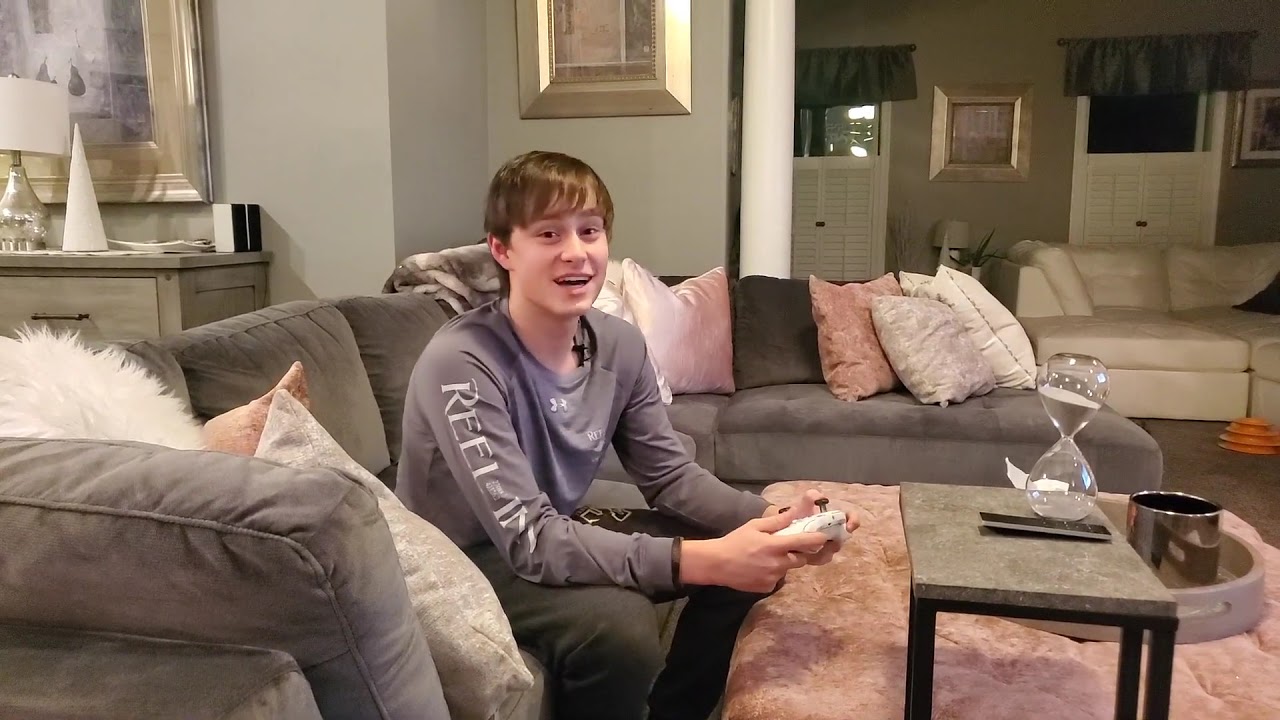In the center of a beautifully decorated living room, a teenage boy with light brown long bangs is absorbed in playing a video game on an Xbox, gripping the controller with both hands and staring intently at the screen. He is dressed in a gray long-sleeve shirt with white text on the sleeve and dark gray pants. The sectional sofa he sits on is a modern L-shaped design in pink, gray, and white hues, with various cushions including a distinctive white fluffy pillow near the armrest.

In front of him, a padded pink coffee table holds an hourglass and a metallic cup resting on the edge of a round tray. A TV remote is also visible on the table, alongside what looks like a dog bed. The backdrop features a stylish living room setting with light gray walls adorned with gold framed pictures, two windows with gray valances, and a white cabinet topped by a silver lamp with a white shade. A conical white sculpture stands next to the lamp, and a small gray wood table behind the sofa holds additional decor, including a couple of black and white blocks.